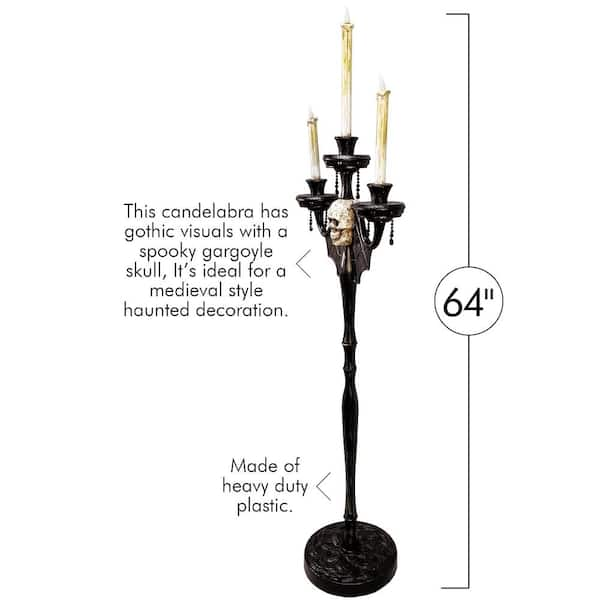This image features a striking black candelabra designed for decorative purposes, possibly for Halloween or medieval-themed settings. Standing at about 64 inches tall, this thin, elongated structure boasts a gothic aesthetic with intricate details. It includes a beautifully engraved circular base that provides stability, and the central column resembles a banister with varying widths, giving it a dynamic look. Dominating the design is a white, smiling gargoyle skull positioned midway up the stem. The candelabra is equipped with three black candle holders, arranged with one atop the skull and two flanking it. Accompanying text describes the candelabra's gothic visuals and confirms it is ideal for medieval-style haunted decorations and is made of heavy-duty plastic, emphasizing its purely decorative function.